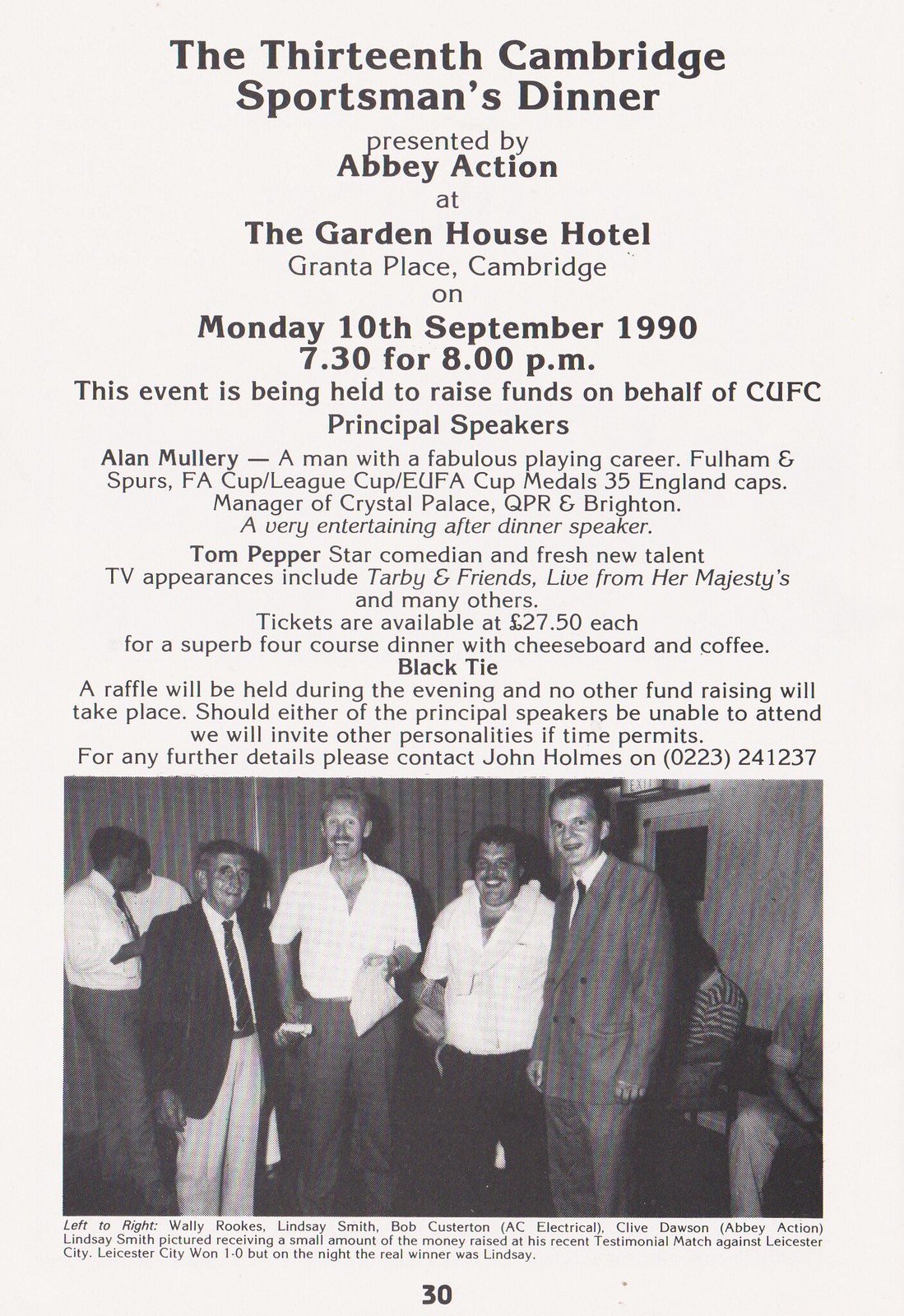This black and white promotional flyer announces the 13th Cambridge Sportsman's Dinner, hosted by Abbey Action at the Garden House Hotel, Grantham Place, Cambridge, on Monday, 10th September, 1990, with doors opening at 7:30 PM for an 8:30 PM start. The event is being held to raise funds on behalf of CUFC Principal Speakers. At the top of the flyer, detailed text provides information about the event, including mentions of notable speakers such as Alan Mullery, an entertaining after-dinner speaker, and comedian Tom Pepper, with brief biographies included. The event promises a superb four-course dinner with a cheese board and coffee, a black-tie dress code, and a raffle. 

The bottom portion of the flyer features an image of attendees, possibly the event hosts or notable figures related to the dinner. In this image, five men stand in a row, all smiling. From left to right, the first man wears a suit and tie; the second, a light-colored shirt and pants; the third, a white shirt; the fourth, another white shirt; and the fifth man wears a gray suit. Some of the men have mustaches, and behind them, other people are seated, suggesting a gathering or meeting setting. The names and details of the pictured individuals are written underneath them, although the text is not fully readable. Overall, the flyer is monochromatic, featuring shades of black, white, and gray, and serves to advertise the upcoming charitable dinner event.